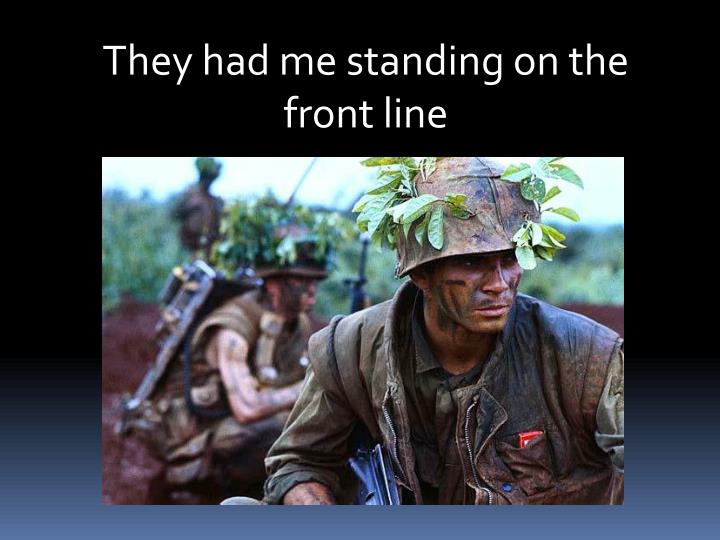The image depicts a color photograph set within a larger, landscape-oriented background that transitions from black at the top to blue at the bottom. Across the top in white text, split over two lines, is the motivational message, "They had me standing on the front line." Below the text is a photograph showing several soldiers in a trench setting during wartime. The soldiers are dressed in dirt-colored camouflage uniforms with additional foliage on their helmets to blend into their environment. One soldier, prominently to the right of the image, is shown from his helmet to mid-chest, holding a weapon under his right arm. His face is painted with camouflage paint, and he wears a brown leather vest over his uniform, bearing a worried expression as he looks to the right. Behind him, two other soldiers in similar attire are slightly out of focus, further enhancing the sense of depth. The background of the photograph includes dark green vegetation and a muddy wall, contributing to the overall realistic and gritty portrayal of trench warfare. The style merges photographic realism with graphic design elements.